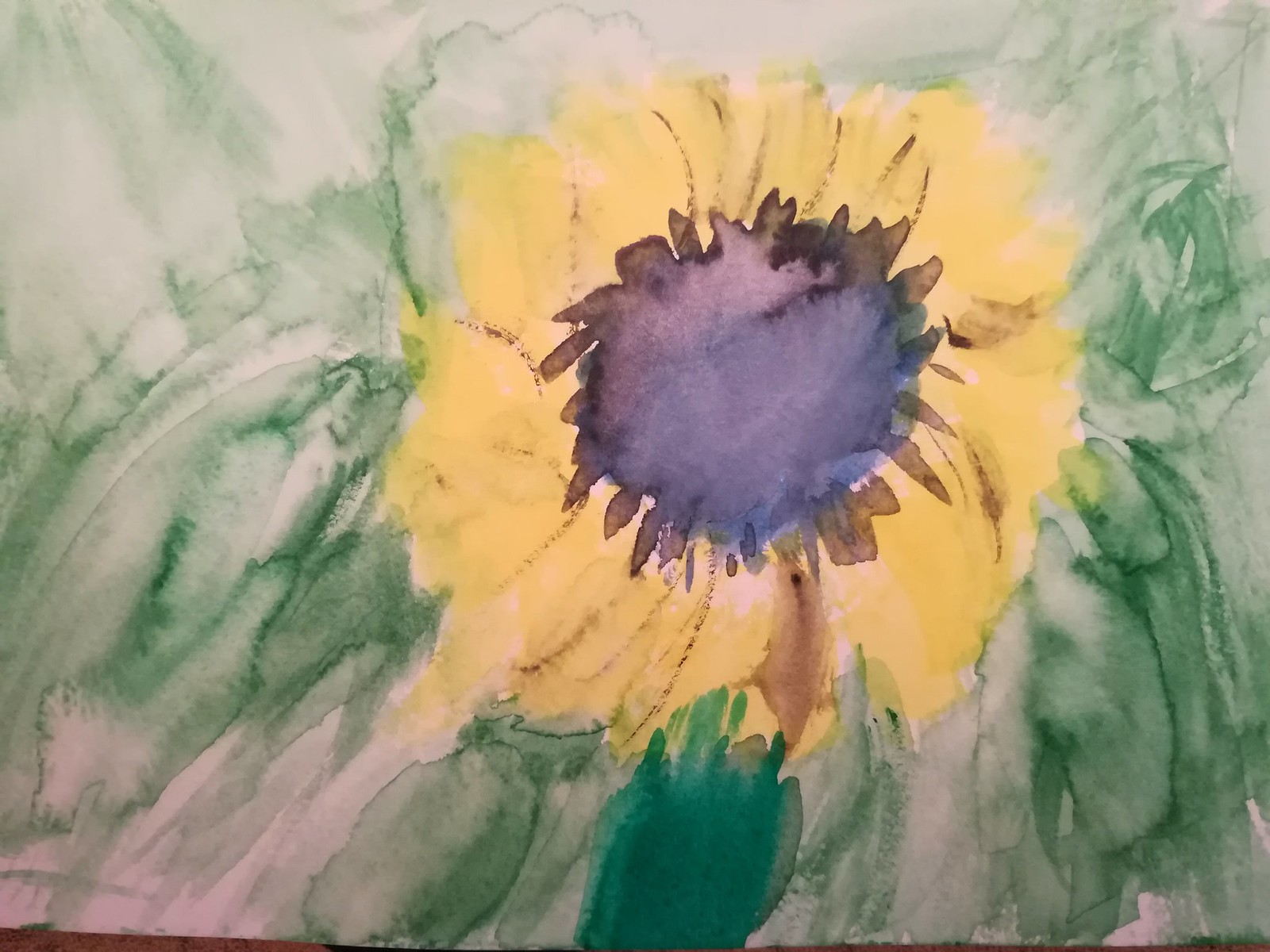This color photograph captures a close-up view of a watercolor painting on a roughly A4-sized white piece of paper, depicting a sunflower. The sunflower, positioned slightly to the right of the center, features vibrant yellow petals with subtle brown streaking to suggest their three-dimensional form. The large central disk of the flower is a blend of purplish-black hues, accented with sporadic black triangular shapes extending around its perimeter. Surrounding the flower are streaks and splotches of varying shades of green, representing the foliage, with lighter greens dispersed on the left, darker tones on the right, and a notable large green splotch at the bottom indicating the stem. The background is largely white, with the greens creating a loose, airy impression of leaves or grass. The painting is unsigned, has no text, and the colors appear somewhat subdued.